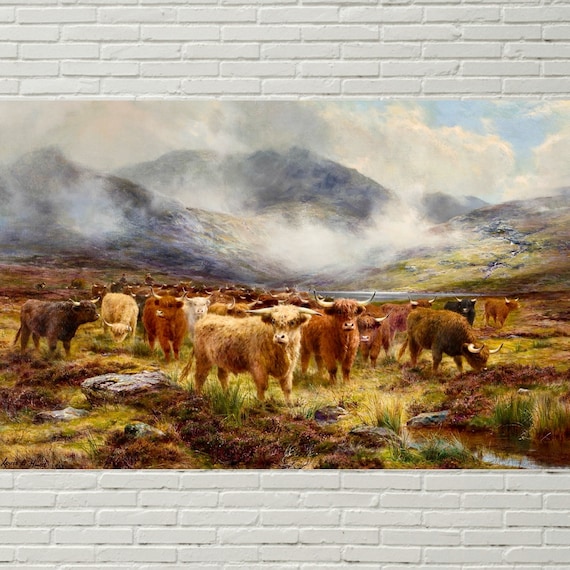The image portrays a painting hung on an off-white brick wall. The painting vividly captures a bucolic scene featuring a diverse herd of roughly 50 to 75 long-haired cattle, including cows and bulls of various shades of brown, black, and white. These cattle, some intently gazing forward, appear to be grazing and meandering in a verdant field interspersed with patches of earthy tones. The serene landscape extends into the background, where fog and clouds obscure rugged mountain peaks. At the base of the mountains, a glimmering river snakes through the scene, adding a touch of tranquility. Above the fog-laden mountains, a sky filled with light blues and scattered white clouds provides a contrasting capstone to this rustic tableau.